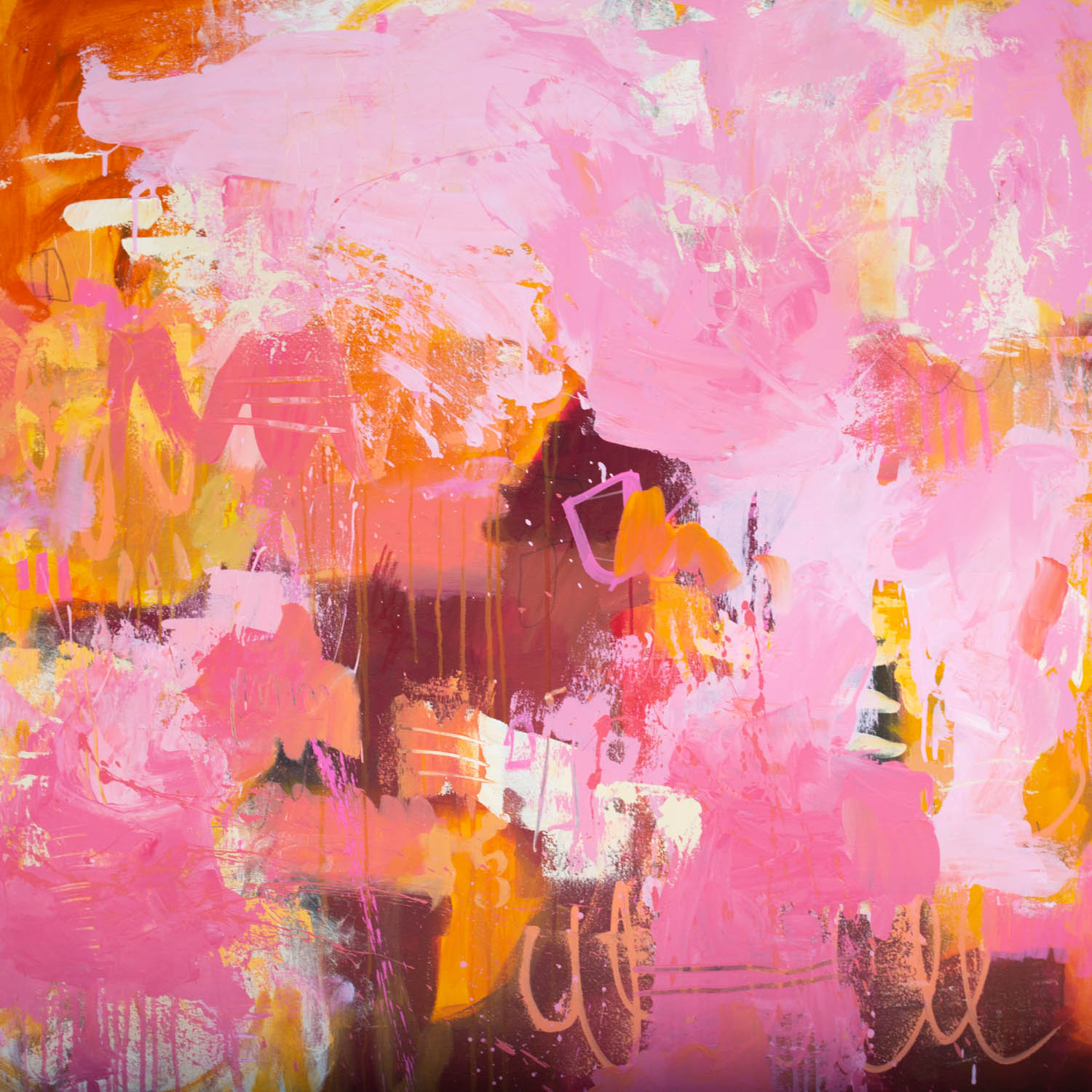The painting, titled "The Game of Life" by Rose Hewartson, is a square-format modern art piece that features an abstract composition dominated by shades of pink, orange, and touches of yellow ochre, white, dark red, and brown. The background is primarily pepto-bismol pink interspersed with light and medium pinks, creating a swirling, collage-like effect. Throughout the painting, there are areas where darker reds and browns blend with gold highlights, particularly toward the bottom left of the center. The top left corner showcases a blend of orange and gold brushstrokes, with erratic white highlights scattered across the canvas. Underneath the complex layers of paint, there appear to be obscured shapes that vaguely resemble people or objects, lending an elusive, almost mysterious quality to the artwork. The bottom right features a light orange scribble that resembles script handwriting but is illegible, adding to the impression of chaotic drizzling paint. This piece is an exemplar of abstract color painting, emphasizing form and color over recognizable shapes or narratives.